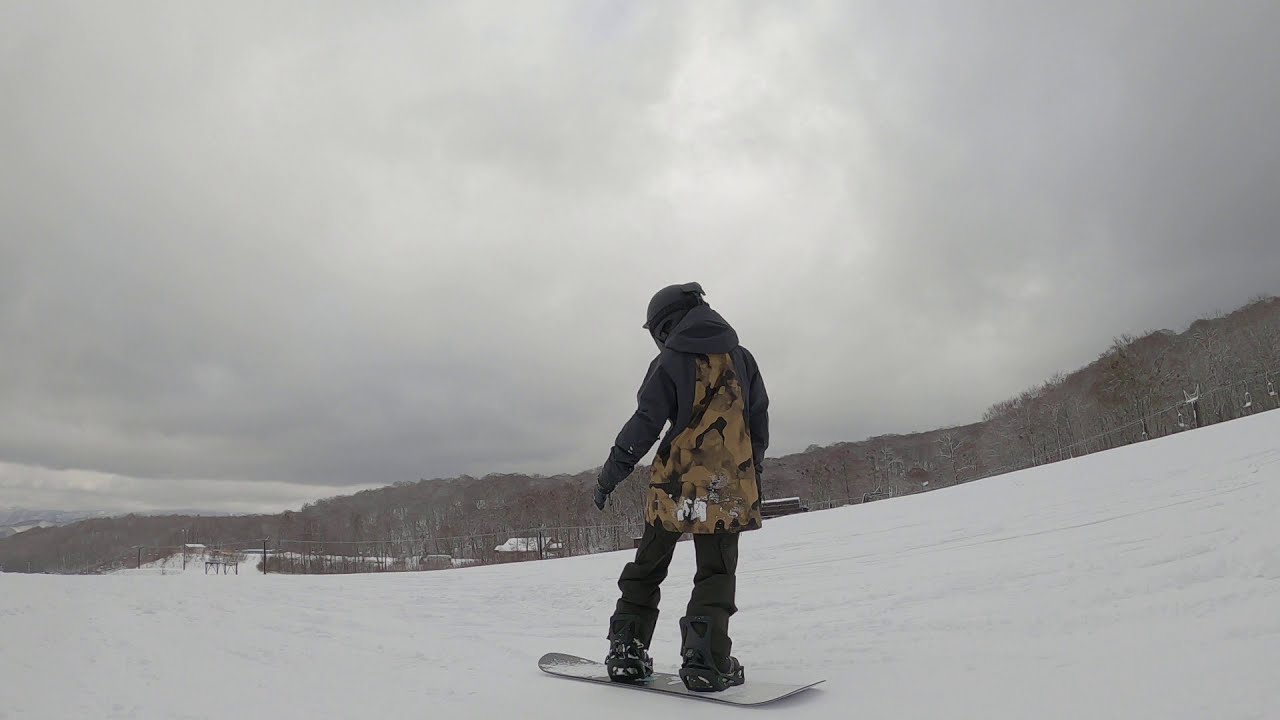This photograph, captured in landscape view, vividly portrays a lone snowboarder descending a snow-covered hill on a bleak, winter day. The snowboarder, appearing youthful, possibly a child, has his back to the camera. He is outfitted in a navy hoodie, black helmet, black pants, black boots, and carries a tan-colored camouflage backpack. Both his feet are firmly planted on a white and gray snowboard. The bottom half of the photo showcases the expansive, pristine white snow.

Above the snowy landscape, winter trees stripped of their leaves stretch across the background, their barren gray-brown branches stark against the wintry backdrop. Adding a sense of depth, ski lift chairs can be faintly seen in the distance. The top third of the image is dominated by a gloomy, overcast sky with heavy, snow-laden clouds, casting a somber and cold atmosphere over the scene. Despite the gloomy weather, the photo captures the serene and solitary essence of snowboarding through a stark, winter landscape.